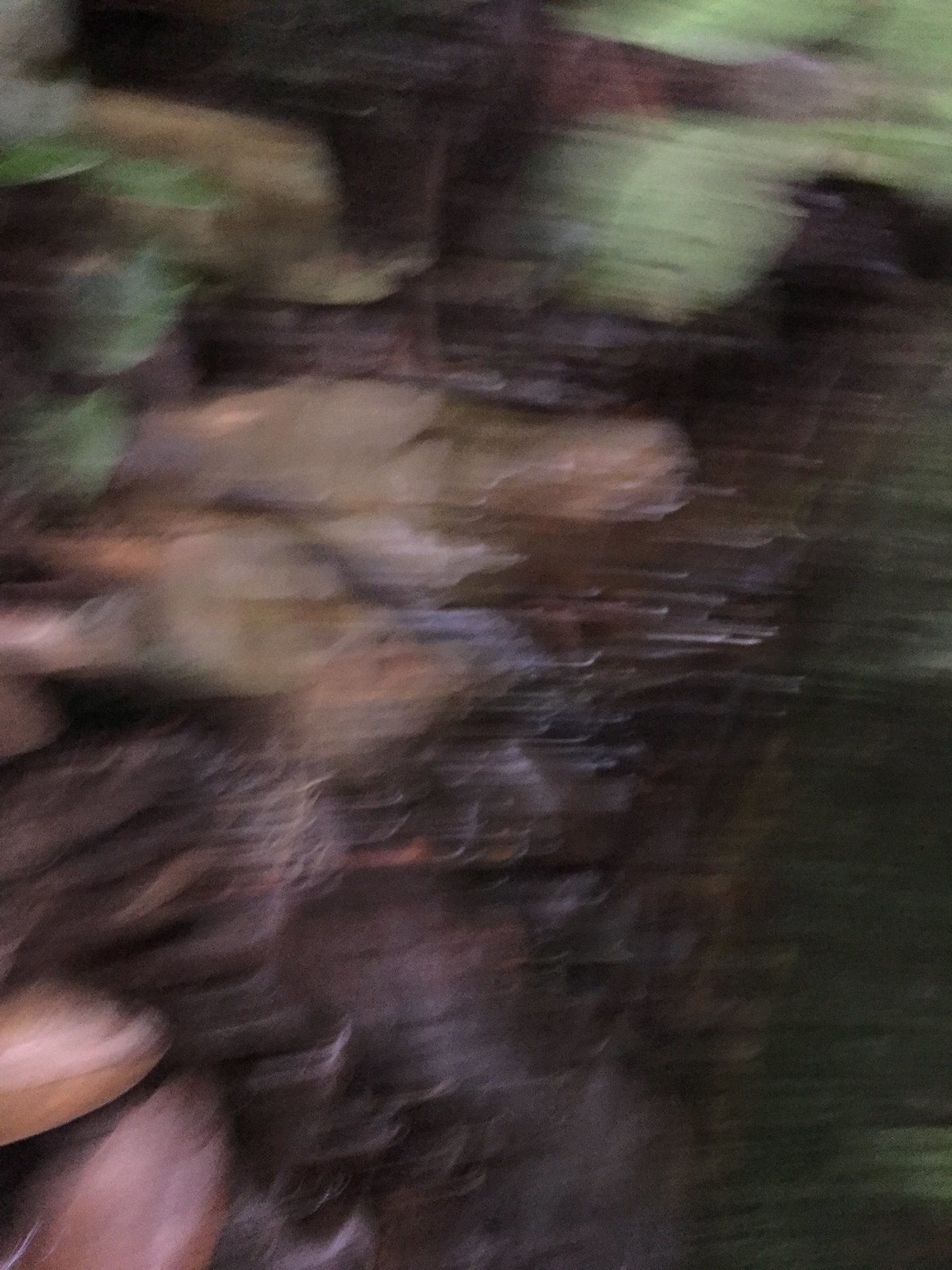This is a color photograph that is vertical and rectangular, characterized by its extreme blurriness, making it almost unidentifiable. The dominant impression is one of vivid, textured colors intermingling without clear designs or forms. The scene is engulfed in a plethora of hues, prominently featuring dark purples with lighter shades in the middle and various streaks throughout. The upper right-hand corner suggests the presence of light green—potentially leaves—while the overall image suggests an earthy or organic backdrop, speculatively like the forest floor with hints of foliage. The conspicuous presence of green shades throughout hints at vegetation, possibly cabbage or broccoli. Additionally, splashes of orange and peach suggest elements like carrots, while lines running through parts of the image add to the mysterious, textured feel. Dark brown patches might indicate mud or dirt, blending with ambiguous blobs of pink and darker, sometimes blackish green areas. Despite the blur, there’s a sense of a layered composition, as if the camera captured a close-up of various organic materials, perhaps a forest floor or a pile of colorful vegetables, rich in texture and complexity.